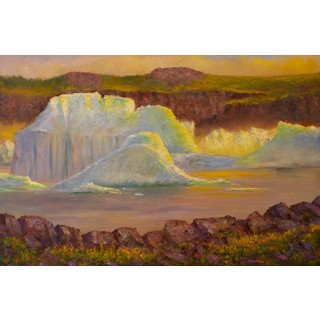The painting depicts a surreal landscape reminiscent of the American Southwest. In the foreground, jagged reddish-brown rocks, rendered with three-dimensional shadowing, lead into a valley filled with formations that strikingly resemble icebergs. These "icebergs" or bright, light-catching rock formations are white with tinges of blue and yellow. Rising through the valley are the tops of mountains or mesas, their white and green summits breaking through a cloud layer. Behind this, an uplifted area of grass features hues of green and red. The horizon showcases an abstract, cloudy sky with muted yet striking colors of yellows and blues. The entire scene is captured in muted, yet vivid tones, which beautifully blend natural and surreal elements.